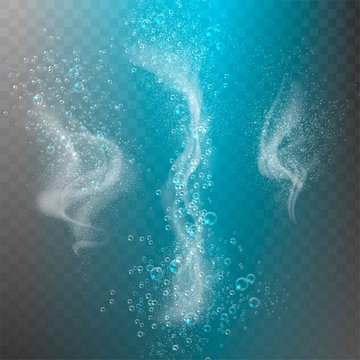The image depicts an underwater scene with a detailed, textured background. The background consists of an alternating check pattern with very small checks that transition from light purple and dark gray on the left, to light blue and dark blue in the center, and finally to dark green and light green on the right. Placed prominently in this vibrant background are three distinct, white, squiggly lines or swirls. The left swirl appears similar to a question mark, emanating bubbles. The central swirl is the most prominent, elongated vertically, resembling a tornado with a bright turquoise hue, and also releasing a multitude of bubbles. The right swirl takes the shape of a 'C' with a tail at the bottom, and like the others, it emits bubbles. There is no text in the image, leaving the visual elements to convey a dynamic and immersive aquatic effect.